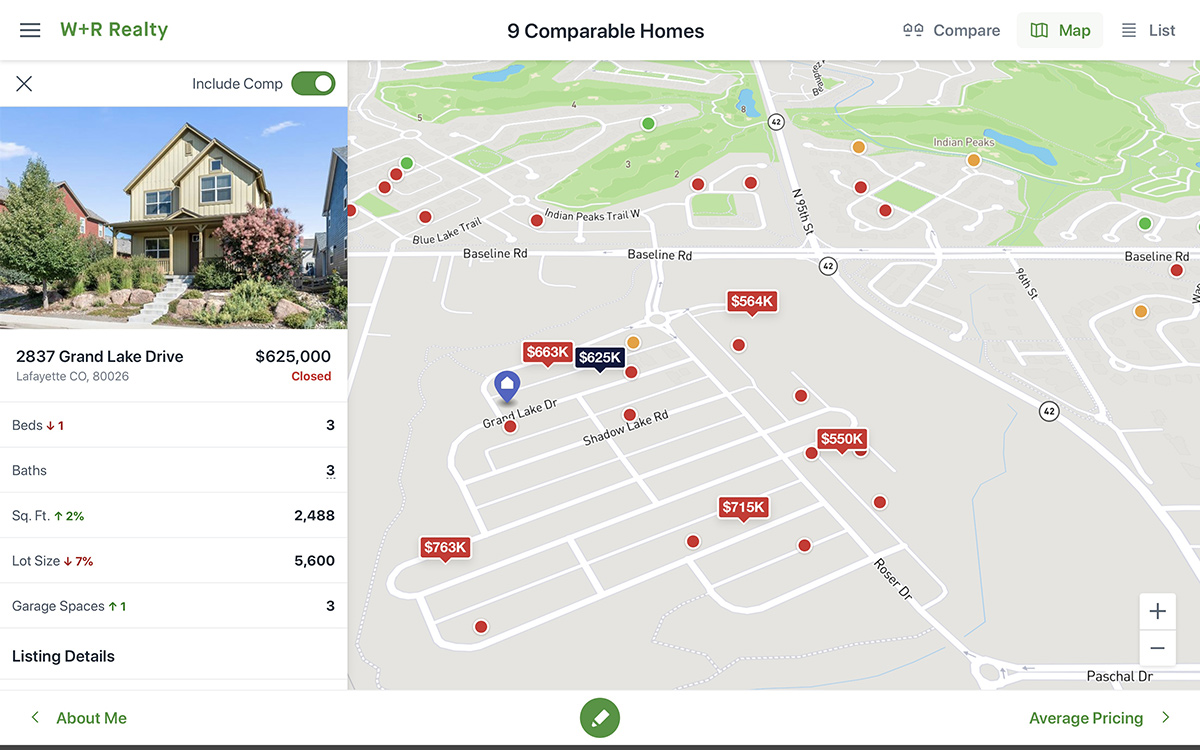This detailed and descriptive caption has been polished and articulated to better depict the content and context of the image:

"In this animation, which resembles a computer screenshot, the top left corner features an icon with three horizontal lines, accompanied by the green text 'W + R Realty.' To the right of this, the text 'Nine Comparable Homes' is displayed, followed further to the right by the options 'Compare', 'Map', and 'List'. Taking up the right portion of the image is a map, depicting white roads, red boxes displaying prices, one black box with a price, and a blue pin marked 'Grand Lake Drive.'

On the left side of the image, there is a photograph of a house with a radiant blue sky in the background. The house itself is a light yellow color, accentuated by a pink tree in the vicinity. The landscape features green shrubs in the front, and leading to the entrance are white stairs. The text adjacent to this picture reads, '2837 Grand Lake Drive, $625,000', indicating the property is located in Lafayette, Colorado.

Beneath this, detailed information about the house is provided: 'Beds: 3, Baths: 3, Square Feet: 2,488, Lot Size: 5,600 sq ft, Garage Spaces: 3'. Further listing details are available, and at the bottom left of the image, there is a green section titled 'About Me.'"